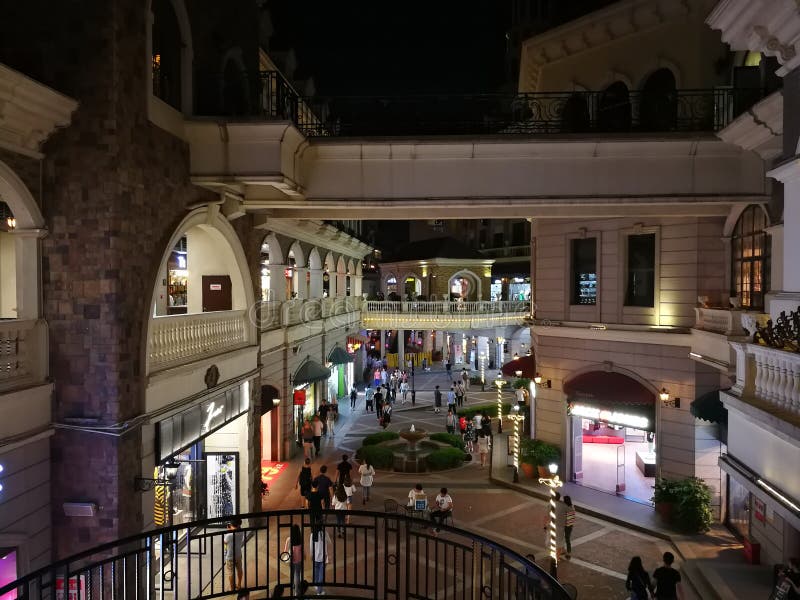A nighttime view from a wrought iron balcony overlooking a charming, European-styled outdoor mall. The shops open into an enclosed plaza adorned with festive decorations in reds and greens. Light poles, wrapped in swirling patterns reminiscent of candy canes, illuminate the scene with subdued yet ample lighting. The ambiance is lively, with people strolling through the area and others seated at tables, enjoying the serene atmosphere. The mall extends into the distance, with streets branching off in multiple directions, inviting further exploration. Offering traditional shops, selling curios and clothing, this picturesque setting feels both inviting and enchanting—a perfect spot for a leisurely visit.